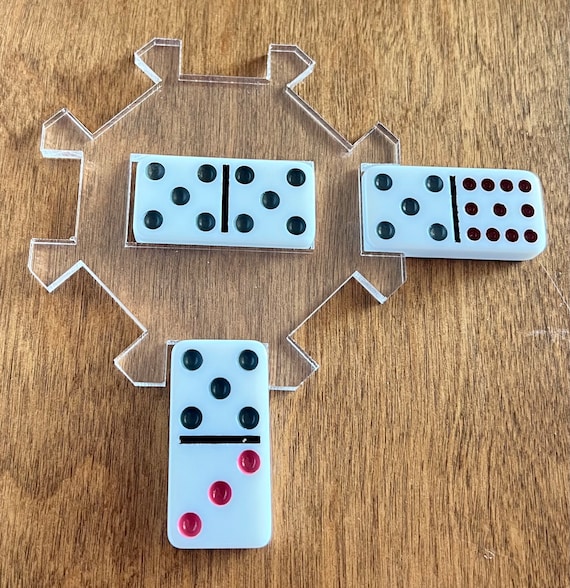In this detailed close-up photograph, three dominoes are prominently displayed on a brown wooden table or countertop. The base domino stands vertically, snugly fitted into a transparent lucite plastic stand that holds the dominoes in place. This vertically oriented domino features a 3 in red and a 5 in black. Positioned above it horizontally is another domino displaying a pair of black 5s. To the right of the center domino, another horizontal one is visible, showing a 5 and a 6 in black. The arrangement and colors of the pips on the dominoes are clearly emphasized against the warm, textured background of the wooden surface.